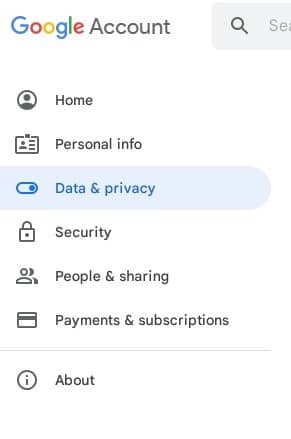A detailed descriptive caption for the image could be:

"Screen capture of a Google Account settings page. The top left corner of the page prominently displays 'Google Account.' A vertical menu on the left is expanded, showing various categories that include 'Home,' 'Personal info,' 'Data & privacy,' 'Security,' 'People & sharing,' 'Payments & subscriptions,' and at the very bottom, 'About.' Each category is accompanied by a corresponding icon to the left: a house for 'Home,' an ID card for 'Personal info,' and so on. The 'Data & privacy' section is highlighted with a blue rectangle, and its text is also in blue, indicating that it is currently selected. The other categories' text remains in black. This visual highlight is designed to draw attention to the 'Data & privacy' settings specifically. To the right of the menu, part of the search bar is visible, with 'Google Account' displayed at the top right corner of the screen. This layout is typical for navigating through the various settings options within a Google Account."